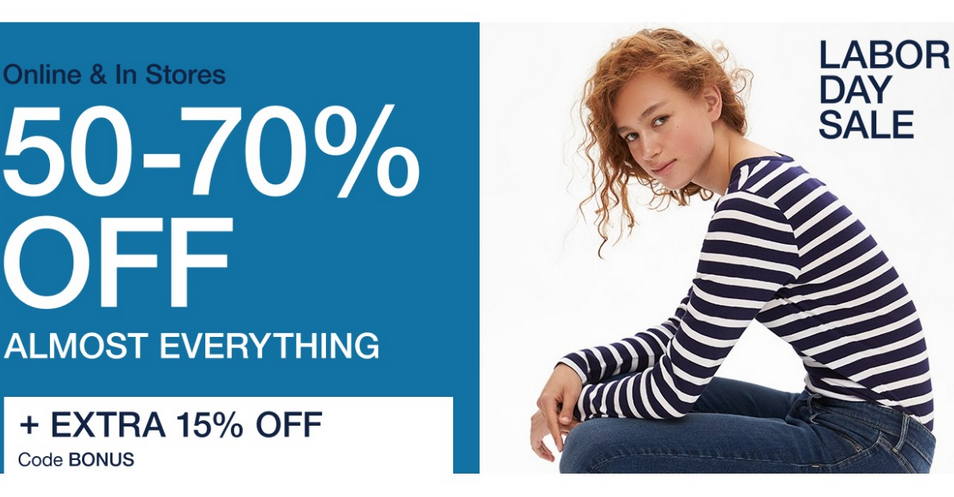Here is the cleaned-up caption with detailed description:

---

The image appears to be a promotional page for a department store, resembling those of retail giants such as JCPenney, Macy's, or Kohl's. On the left side of the page, against a blue background, white and blue text announces an enticing offer: "Online and in stores: 50 to 70% off almost everything, plus an extra 15% off with code BONUS." 

To the right, the visual features a model donning a stylish outfit. She is seated and facing left, with her head turned slightly towards the camera. Her ensemble includes blue Levi's jeans and a white and navy blue long-sleeve shirt. The model has curly red hair, adding a dynamic touch to the scene. In the upper right-hand corner, "Labor Day Sale" is prominently displayed in dark blue text, anchoring the promotional theme.

---

This caption provides a detailed and clear description of the promotional image.